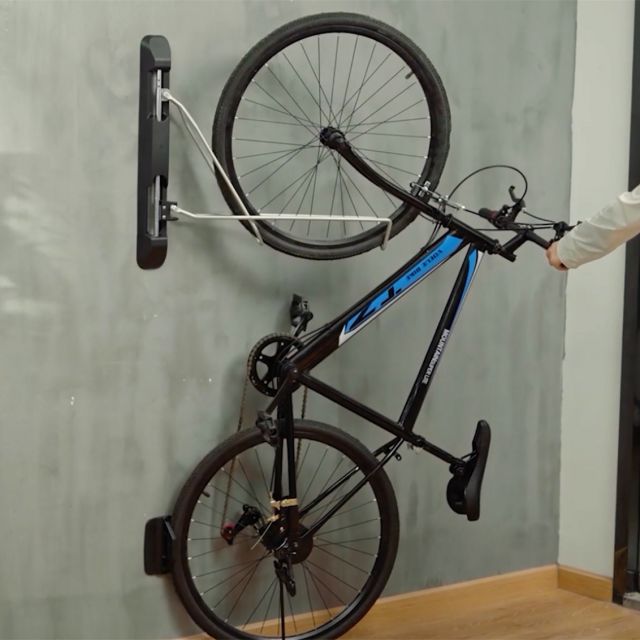This photograph features a bicycle mounted on a gray wall, though it initially appears as though the image might be oriented incorrectly, suggesting the bike could be on the floor if the photo were rotated. The bicycle's back wheel is securely fastened to the wall with a visible mounting device. The bike's frame is predominantly black with a striking, contrasting blue section. Near the front wheel, there's a long rectangular gray object, possibly part of the mounting or display system. Additionally, two gray cables are visible, attached to the front wheel, adding to the complexity of the scene. In the bottom right-hand corner, we see a segment of brown hardwood floor, along with a matching baseboard, indicating this photo was taken at a corner of a room. The combination of these elements creates a perplexing and intriguing visual.